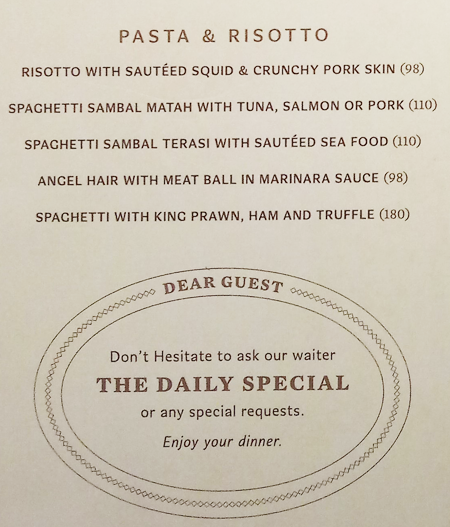The section of this menu presents a selection of pasta and risotto dishes in a well-organized format. Printed on an off-white, aged-looking rectangular background with dark brown, capitalized text, the header reads "PASTA & RISOTTO," centered at the top.

The first dish listed is "Risotto with Sautéed Squid and Crunchy Pork Skin (98)," followed by "Spaghetti Sambal Matah with Tuna, Salmon, or Pork (110)," "Spaghetti Sambal Terasi with Sautéed Seafood (110)," "Angel Hair with Meatball in Marinara Sauce (98)," and "Spaghetti with King Prawn, Ham, and Truffle (180)."

The bottom half of the menu features an ornate oval design with the text centered inside. It reads, "DEAR GUESTS," followed by "Don't hesitate to ask our waiter the daily special," with "DAILY SPECIAL" in bold capitals. Beneath that, it states, "Or any special requests" in italics, and concludes with "Enjoy your dinner."